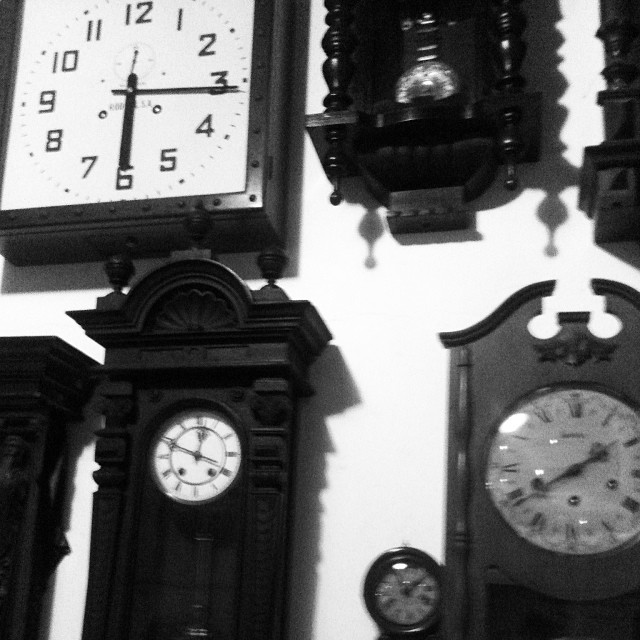The black and white photograph showcases an array of clocks mounted on a pristine white wall, casting faint shadows that add depth. In the top left corner, a prominent square clock with a black frame and white face features classic black numerals from 1 to 12, indicating a time of 6:15 with its long, slender, and fat black hands. This clock's borders extend beyond the frame of the photograph. Beneath it, a partial view of a dark, chime-like clock can be seen, reminiscent of a diminutive grandfather clock, with a slender, hanging pendulum. Moving right, a stately rectangular clock resembling a grand building captures attention with its domed top accentuated by little gray squares and three black knobs. The white clock face set centrally shows black Roman numerals and sleek black hands. Further down, on the lower left, a faint outline of another black clock barely peeks into the shot. Adjacent to it, a blurry, small round clock adds to the vintage ambiance. Lastly, a distinctive tall rectangular clock, rounded at the top with intricate cutout designs and a black border, stands proudly, completing the eclectic mix of timepieces that evoke a sense of nostalgia and collectors' pride.